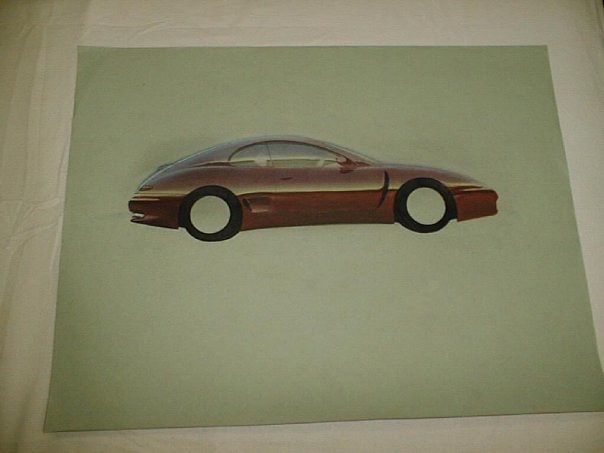This image showcases an artistic illustration, possibly created by hand or digitally, of a sleek two-door sports coupe that closely resembles the style of a Porsche. The car features a muted burgundy, almost maroon color, and a distinctive yellow line running down the middle. The wheels have black tires with stark white centers where the rims would typically be, but there are no spokes. The illustration is set on a green piece of paper, which serves as the canvas. Behind this green sheet, there is a white background, which could be a piece of cardboard or a bed sheet, adding to the layered, textured presentation of the image.